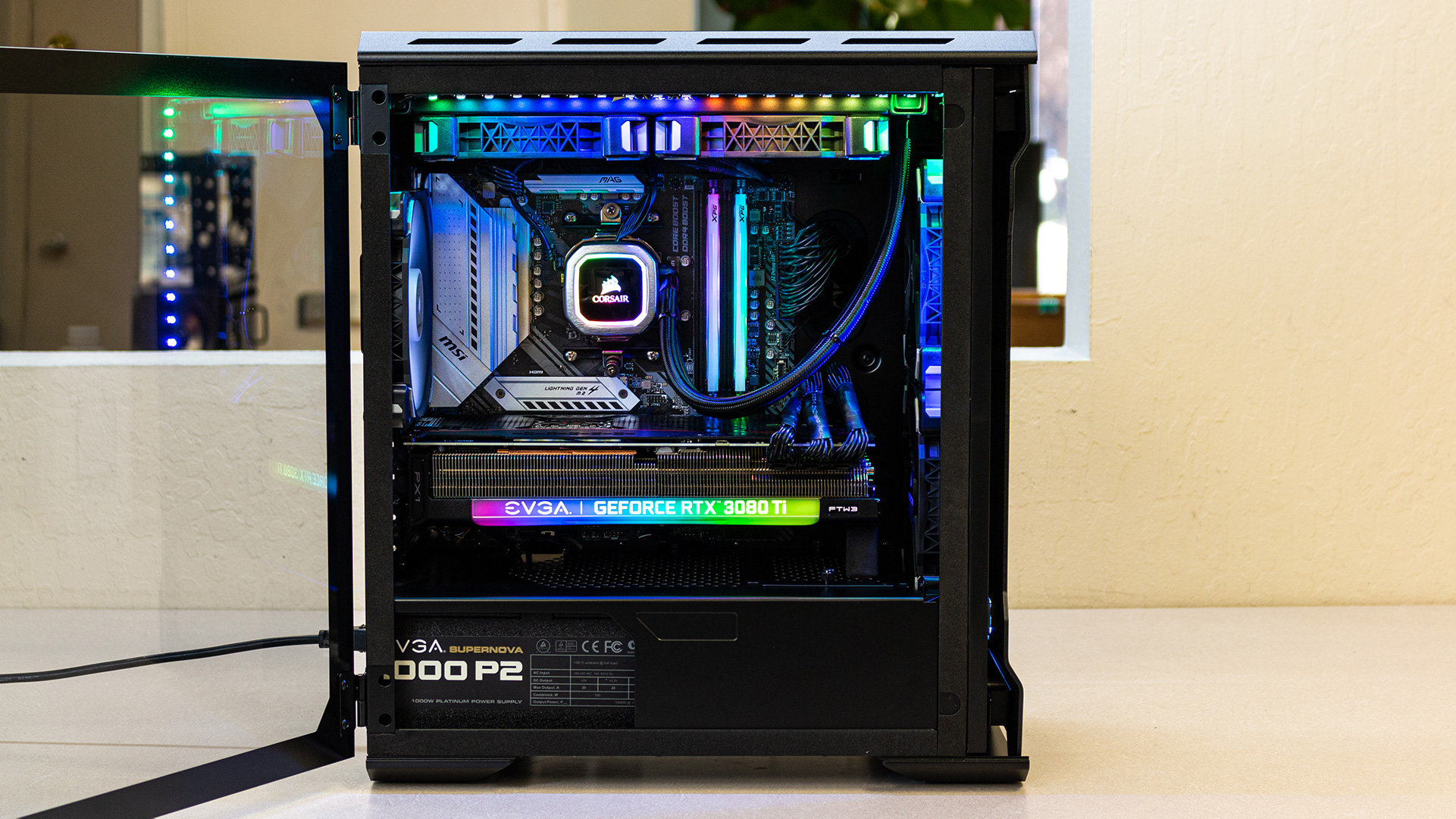The photograph showcases a tall, powerful custom-built gaming computer with an open black case resembling a small cabinet with glass doors. Inside, a dazzling array of multicolored lights illuminate the components, featuring hues of green, blue, light blue, purple, red, and yellow, creating a rainbow effect. Prominently displayed on the hardware is the label "GeForce RTX 3080 Ti," indicating the presence of a high-end graphics card, with additional labels such as "EVGA" and "Supernova" visible on various parts. The interior reveals a complex arrangement of wires, tubing, and circuit boards, suggesting a meticulously assembled machine. The setup rests on a white surface against a backdrop of beige walls, with hints of another room and a door in the distant background.